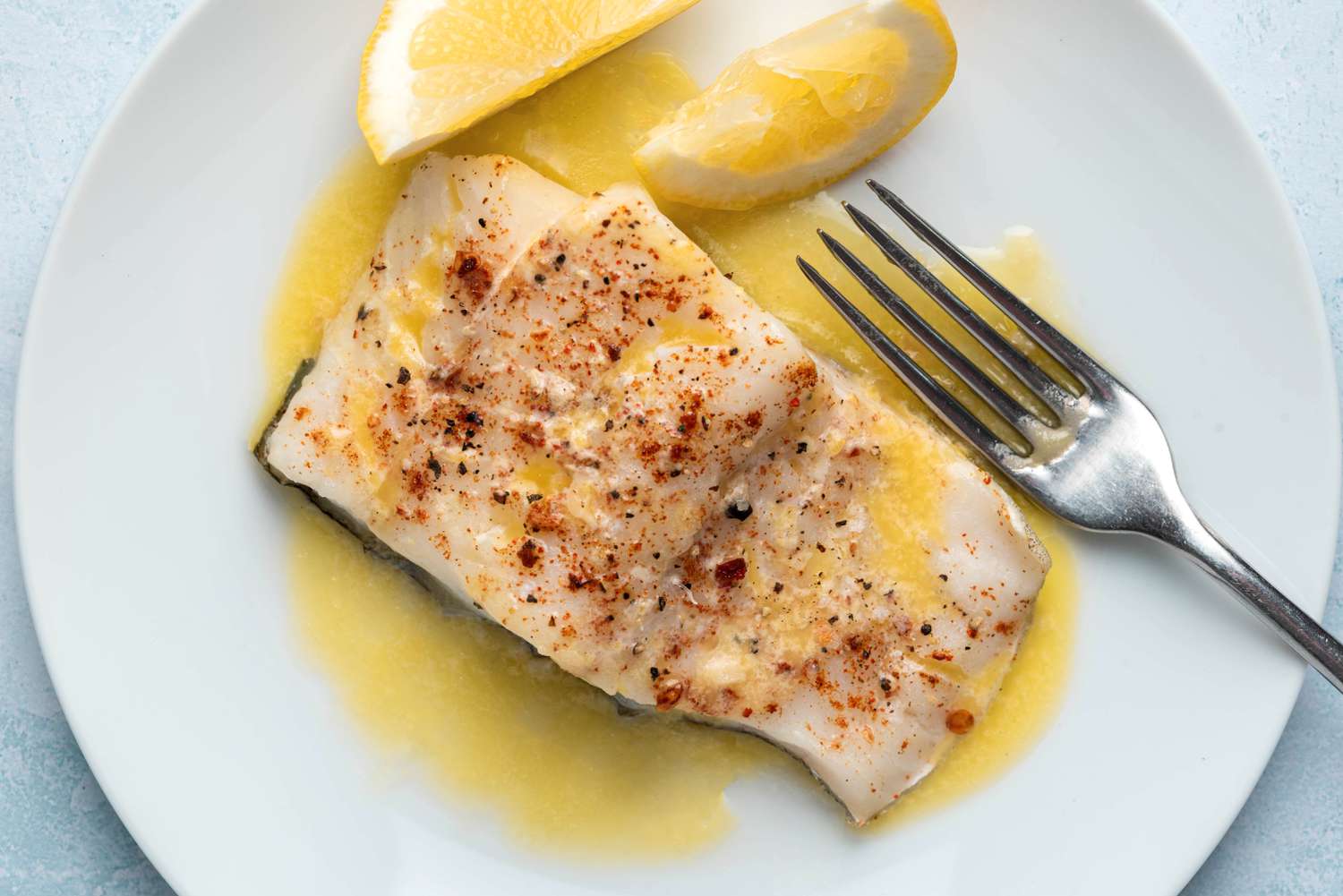The photograph showcases an appetizing dish, ideal for a recipe website. Centered on a white plate set against a marbled white countertop, the dish consists of a seasoned piece of fish, possibly salmon, displaying a flaky texture. The fish, with its lightly pink and white hues, is generously sprinkled with paprika and other spices, resting on a bed of yellow sauce that might be butter. The dish is garnished with two lemon wedges at the top of the plate, one of which is upright on its rind. A dark edge of the fish's skin is subtly visible along the bottom. To the right of the plate, a silver fork lies slightly dipped into the yellow sauce. The overall composition features a harmonious blend of whites, off-whites, yellows, and a vibrant splash of red from the paprika, delivering a visually appealing and mouth-watering presentation.